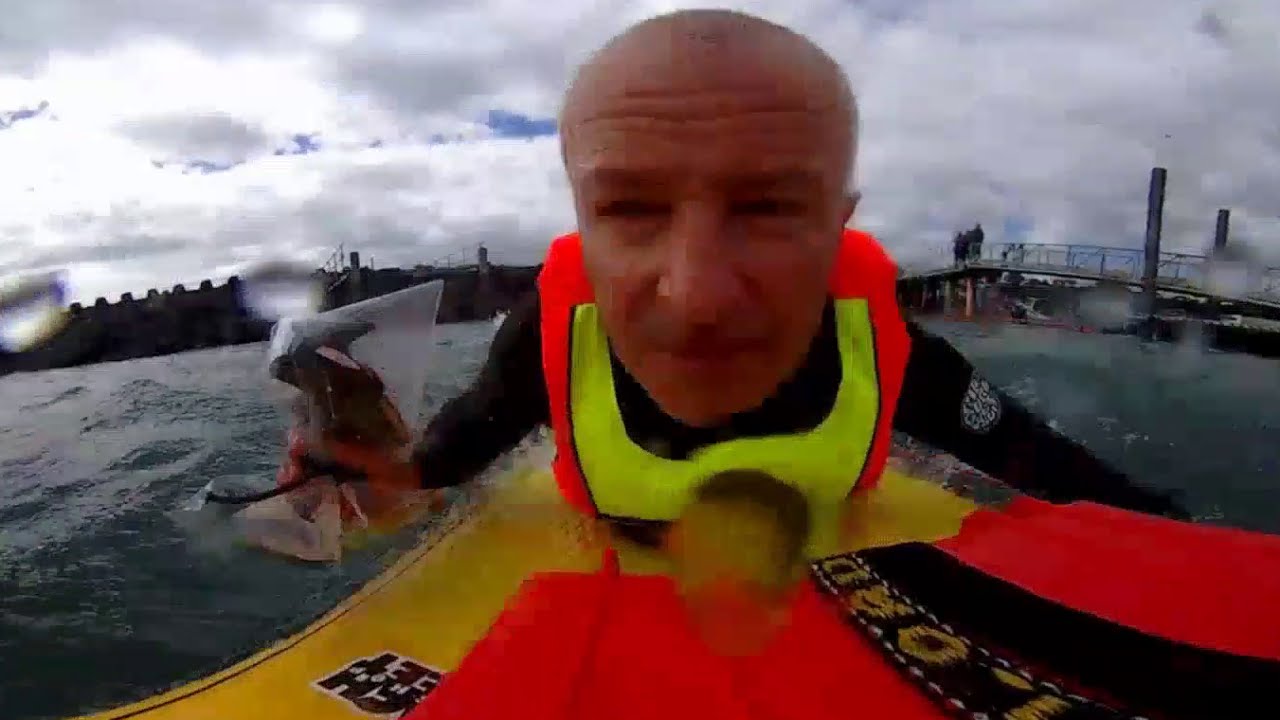The photograph, though pixelated and slightly out of focus, captures a bald man around 50 years old on a neon orange and yellow surfboard, wearing a fluorescent lime green, black, and orange life vest over black long sleeves. The man is paddling on his stomach, looking directly at the camera. The yellow surfboard features illegible text on its yellow portion, and the word "L-O-R-D" can be discerned on its orange section. An indeterminate object with black and red tones floats nearby to the right of the man. The background reveals a choppy ocean, with a metal bridge on the right and a dark silhouette of a wall forming a jetty on the left. The sky above is a mix of blue and gray with prevalent clouds, suggesting an overcast day. The image appears to have water droplets on the lens, hinting at recent splashes during the photograph capture.